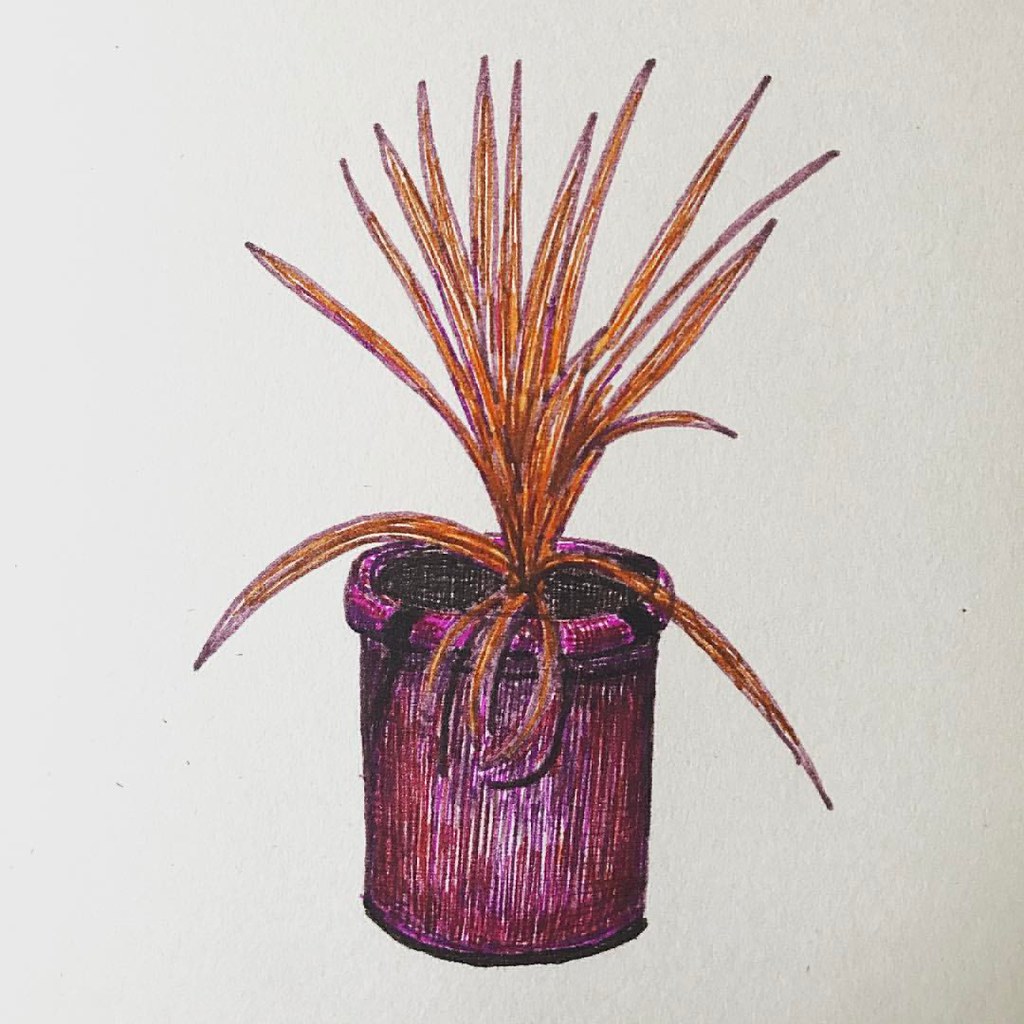The image showcases a detailed pen drawing with a grey background, featuring a round, purple flower pot characterized by an intricately drawn rim at the top and a black interior. Emerging from the pot is an orange plant with numerous straight stalks, reminiscent of monkey grass but distinctly colored. A few of the plant's stalks bend gracefully over the edge of the pot. The illustration employs a technique where lines are meticulously drawn to create texture and depth, leaving intentional white spaces throughout the composition for a dynamic, partially-filled visual effect.